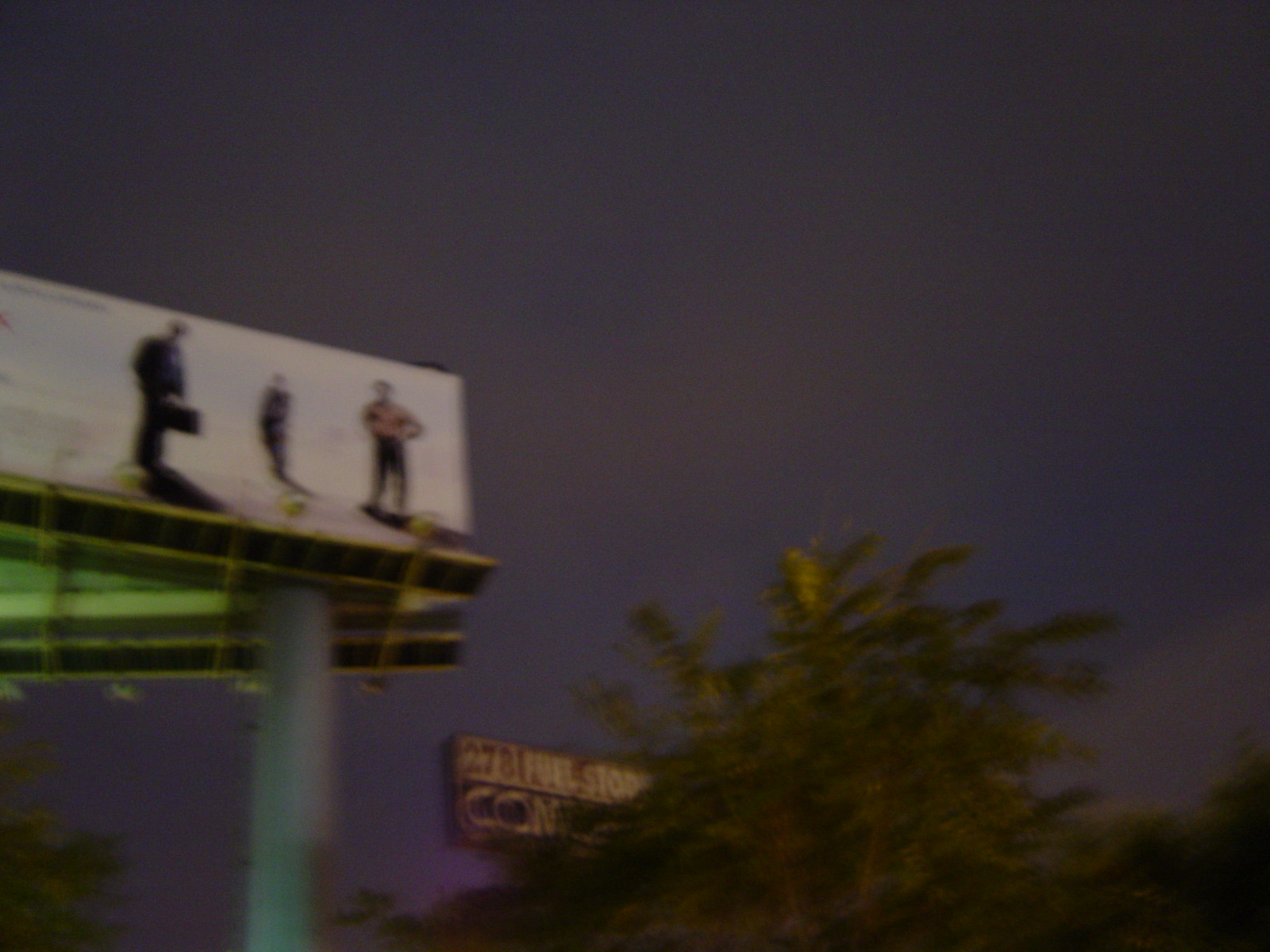A large billboard towers high above the surroundings, displaying a blurred advertisement featuring three individuals. On the right, a man dressed in brown pants and a pink shirt stands confidently. The center figure, also clad in brown, has an indistinct appearance. On the left, another person, dressed in blue, holds a suitcase or briefcase. Behind this billboard, only the green backing of another advertisement is visible. The billboard surpasses the height of a nearby palm tree, which has one yellowish, discolored frond among its otherwise green leaves. Additionally, the billboard rises above another advertisement marked by red, white, purple, and yellow colors. The sky in the background appears ominous, suggesting an approaching storm as darkness begins to settle in.